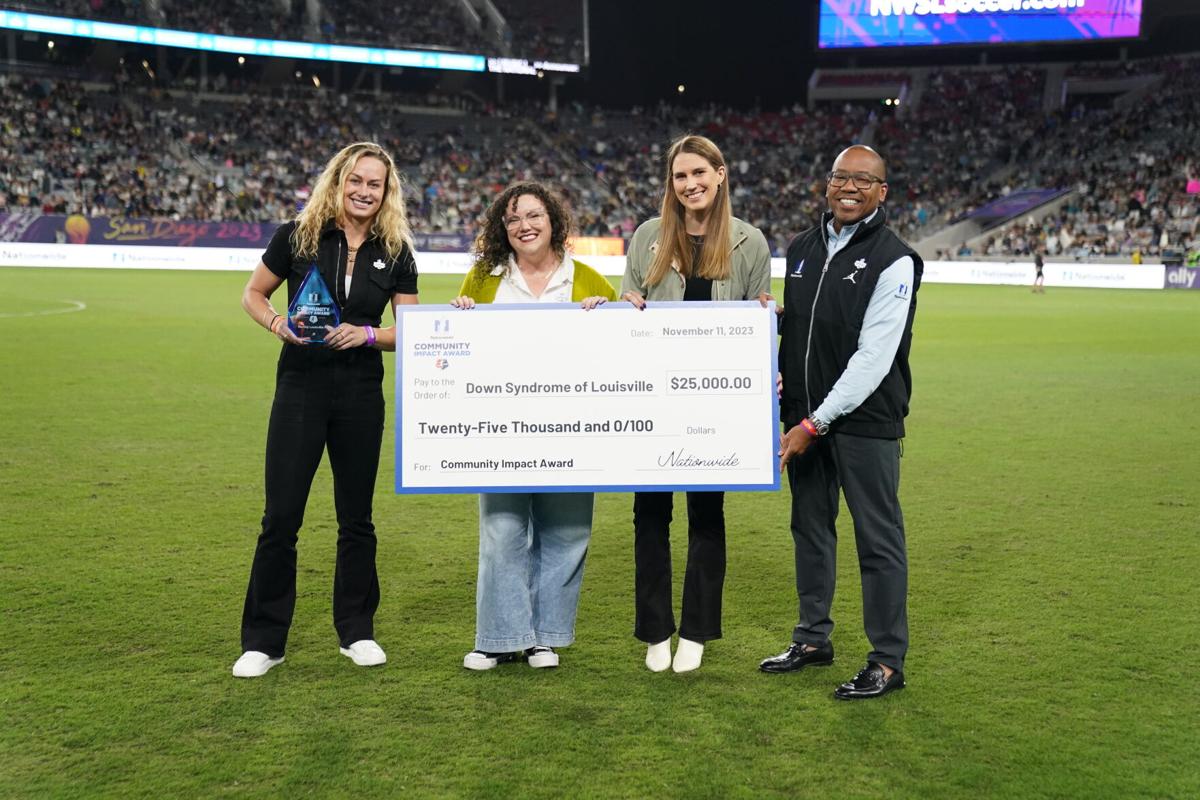This is a nighttime photograph of four people – three women and one man – standing on a grassy sports field with filled spectator stands in the background. They are gathered for a presentation, possibly during an athletic event, holding a giant promotional check. The check, white with a blue border, is made out to Down Syndrome of Louisville for the amount of $25,000 and is dated November 11th, 2023. It bears the title "Community Impact Award" along with a Nationwide logo. The woman on the left, dressed in all black with long blonde hair, is holding a triangular blue and white crystal trophy. The group appears very happy, celebrating the significant donation.